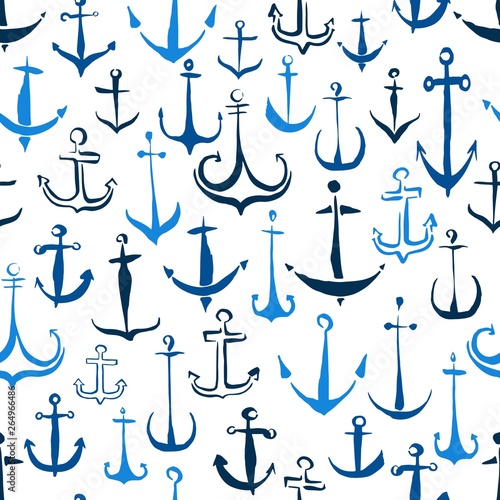This image features a vibrant and meticulously arranged graphical pattern of various artistic renditions of anchors against a pure white background. The anchors come in different shades of blue, ranging from deep dark blue to very light blue, and alternate in color as they are arranged approximately in rows, covering the entirety of the background. They are slightly offset, creating a dynamic elevation that adds depth to the pattern.

The designs of the anchors vary widely, with some capturing the basic shape with a simple circle, a line, a cross line, and a V-shaped bottom, while others are more elaborate with curved forms, arrows, and bulbous tops. Some anchors are just outlines, demonstrating a range of artistic interpretations from minimalist to intricate. 

Additionally, on the left-hand side of the image, there is a vertical inscription that reads "Adobe Stock 264966486," indicating that this is an Adobe-branded graphic. The overall effect is reminiscent of a stylish patterned fabric or wallpaper, showcasing an array of blue-toned anchors in diverse forms and styles.